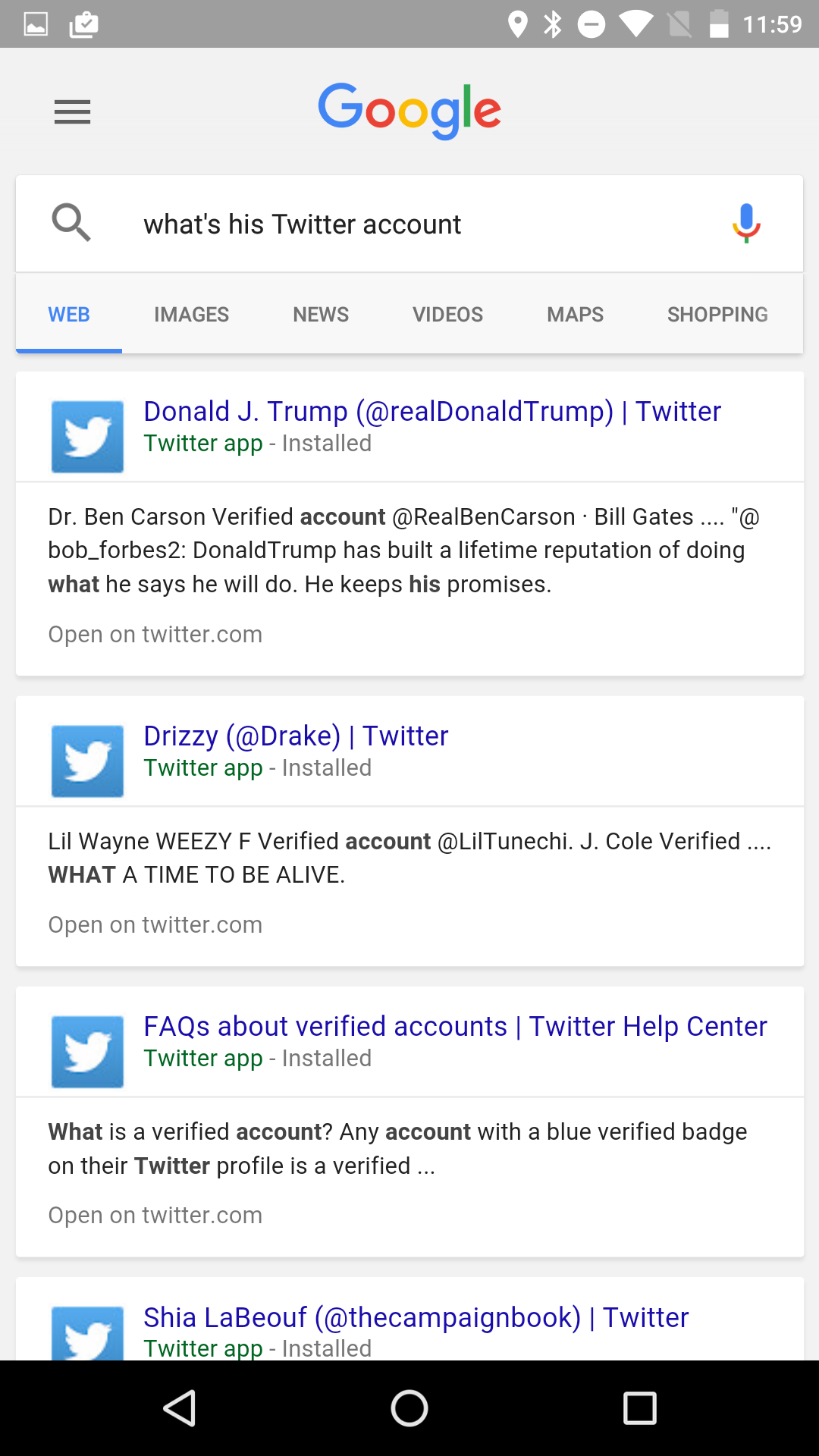The image captures a screenshot of a Google search query. At the top center of the screen is the Google logo, followed by the search bar where the user has typed "what's his twitter account." Below the search bar are several category options: "All," which appears in blue text and is underlined, indicating it is the currently selected category, followed by "Images," "News," "Videos," "Maps," and "Shopping."

The search results begin with the first listing: "Donald Trump (@realDonaldTrump) on Twitter." The second result is "Drizzy (@Drake) on Twitter," followed by the third result, a FAQ entry titled "About Verified Accounts – Twitter Help Center." The fourth and final visible listing partially displays "Shia LaBeouf - The Campaign Book on Twitter." Along the left side of each result is a small blue square icon containing the original white Twitter bird logo. Beneath each result appears some snippet text, likely posts from the corresponding Twitter accounts.